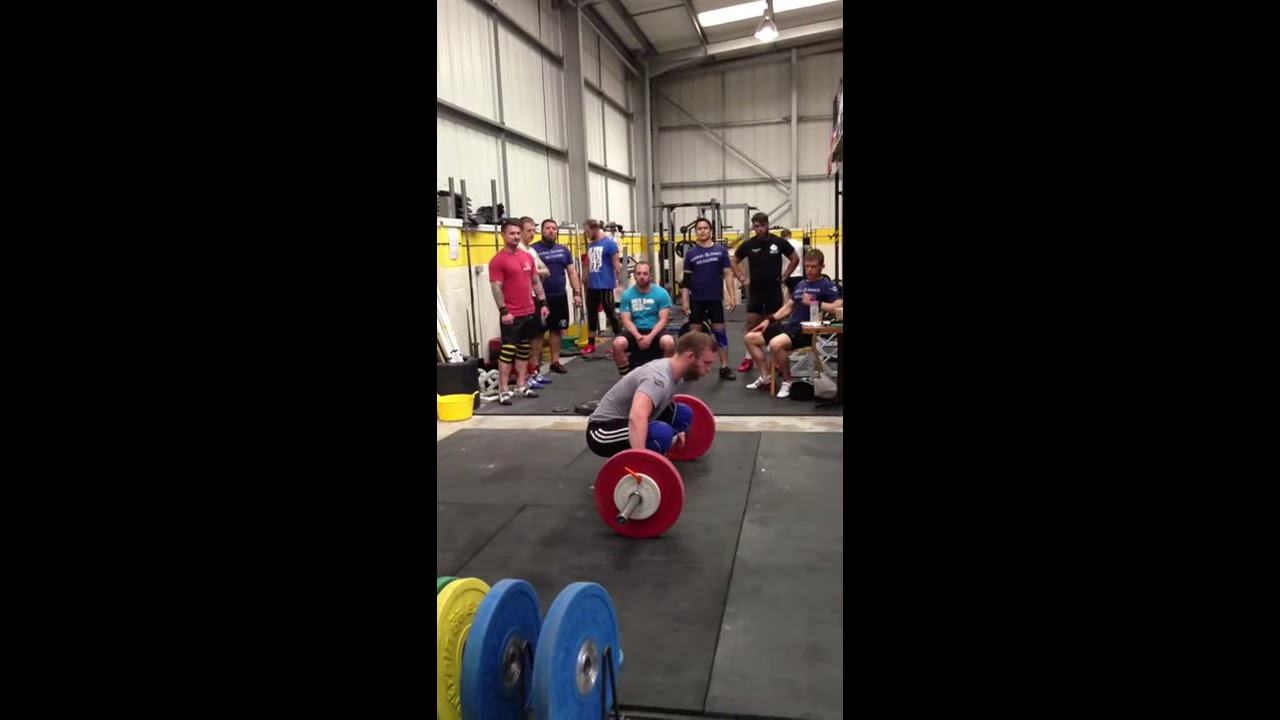In the center panel of a triptych with black bars on the left and right, a vertically aligned photograph captures a scene inside a high-ceilinged, metal-walled gymnasium. The focal point is a bearded Caucasian man, likely in his early 20s, poised mid-squat as he prepares to deadlift a barbell adorned with red weights. He is outfitted in a grey t-shirt and blue pants with white stripes, standing on a black cushioned mat. Surrounding him are several similarly dressed young men, mostly wearing t-shirts and shorts, with a few notable colors like blue, aqua, and red among them. These onlookers, who are either standing or sitting, seem intently focused on the lifter, suggesting an event of significance such as a personal record attempt or an informal competition. The gym is fully equipped with numerous weight racks and mats, indicating a dedicated weightlifting environment. The overhead lighting and a skylight illuminate the area, casting light over the scene where the only visible text is minute and unreadable on the t-shirts of the spectators.